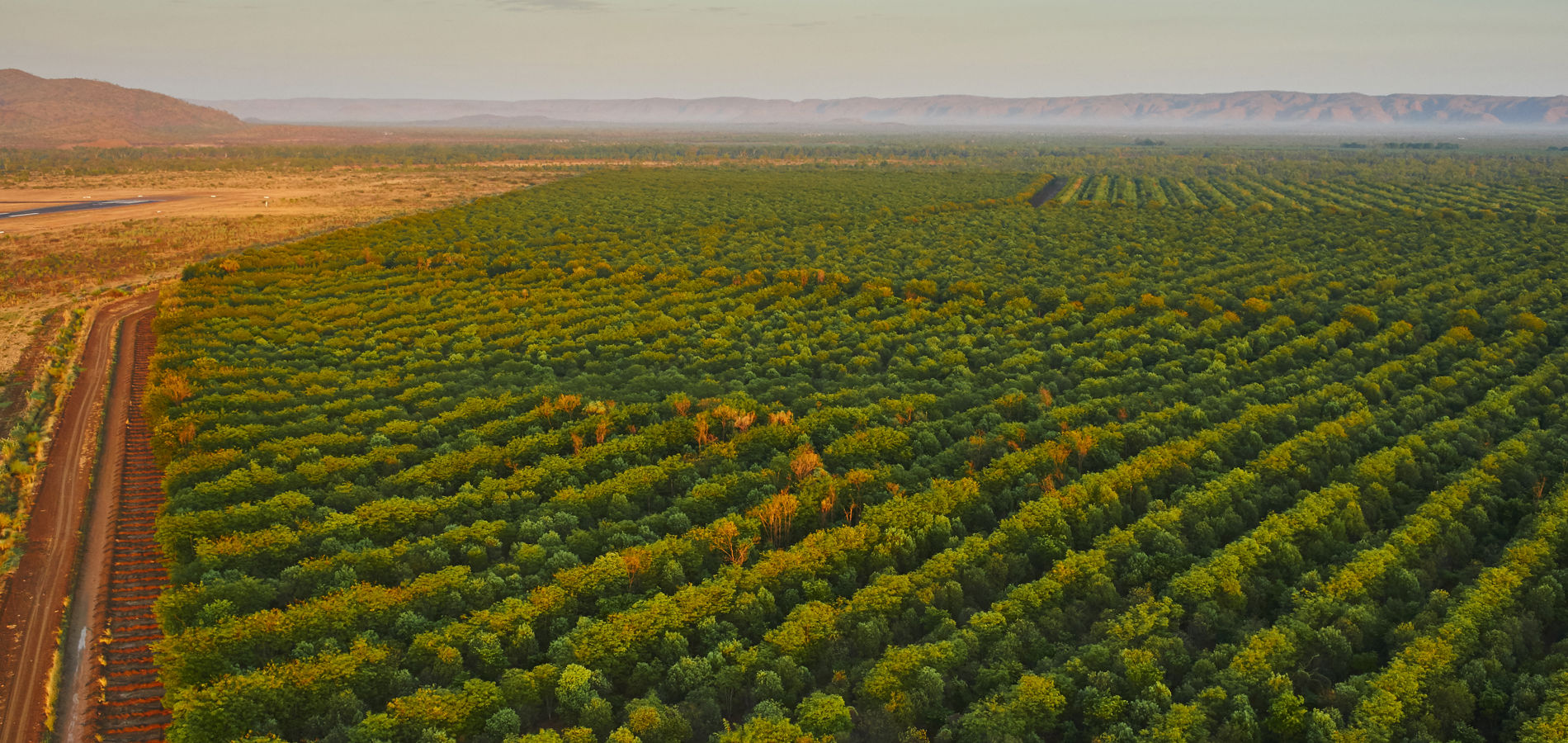An aerial photograph captures an expanse of farmer's fields and groves of tall, bushy trees arranged in meticulous rows, predominantly green with patches of yellowed, less healthy plants. The scene indicates an arid region with the vibrant fields contrasting against the surrounding dry, brown soil. The fields are subdivided into regions with rows running in various directions, potentially for erosion control. On the left, a muddy brown path, marked by vehicle tracks, weaves through the landscape. In the far distance, a series of brownish, orangish, and reddish mountains rise, with some hazy fog adding depth to the background. The entire scene is a testament to the organized cultivation and agricultural use of the land, set against the dramatic backdrop of mountainous terrain.